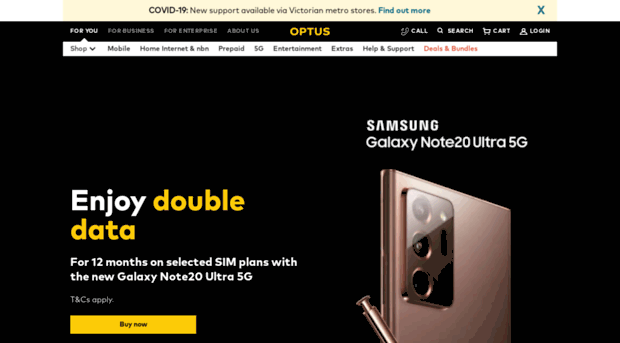The image showcases a webpage with a sleek black background. At the very top, there is a prominent yellow rectangular banner that reads: "COVID-19. New support available via Victorian Metro Stores. Find out more." accompanied by an X button for closing the message. Below this header, the majority of the background remains black.

On the bottom right of the image, an elegant rose gold Samsung Galaxy Note 20 Ultra 5G is displayed, featuring three rear cameras and a gold stylus. The device is highlighted by a caption above it in white text stating "Samsung Galaxy Note 20 Ultra 5G."

To the left of the phone, there is a promotional message: "Enjoy double data," with "double data" emphasized in yellow, followed by "for 12 months on selected SIM plans with the new Galaxy Note 20 Ultra 5G. T&Cs apply." Directly below this promo, a yellow button with black text invites users to "Buy Now."

At the very top of the page, there is a navigation menu with various sections. The currently selected section is "For You," while other options include "Shop" with a drop-down arrow, "Mobile," "Home Internet," "NBN," "Prepaid," "5G," "Entertainment," "Extras," "Help and Support," and "Deals and Bundles." Additional sections for "Business," "Enterprise," "About Us," "Optus," "Call," "Search," "Cart," and "Log In" are also visible.